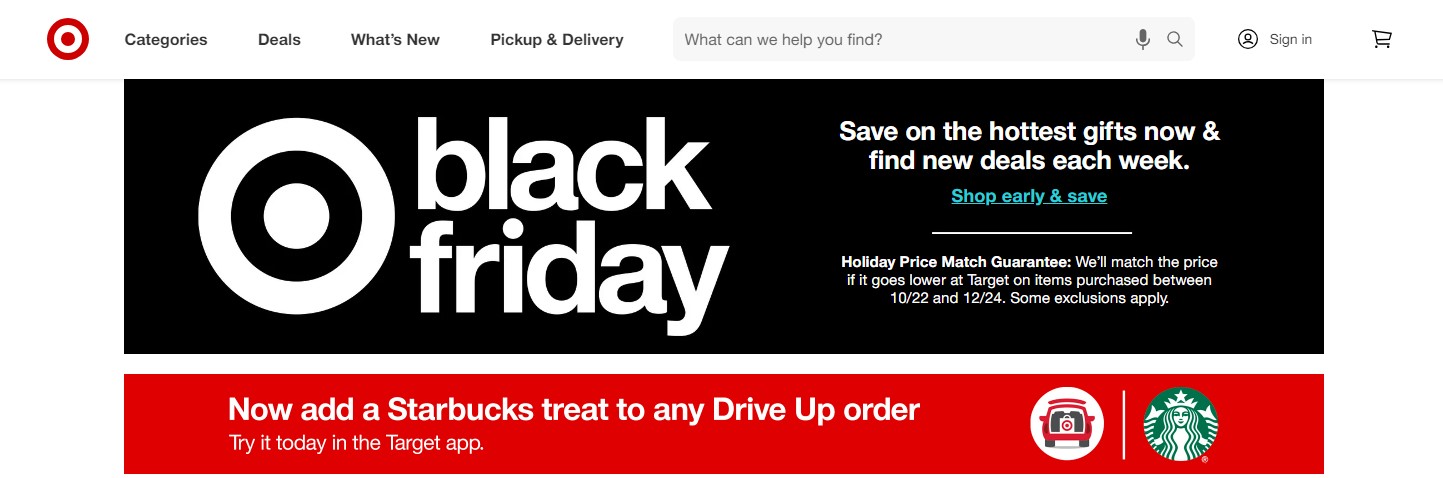This is a detailed screenshot from a Target website. The top section features a prominent white bar on the left corner displaying the iconic Target logo, a red circle with a red dot in the center. Adjacent to the logo are clickable menu entries titled 'Categories,' 'Deals,' 'What's New,' and 'Pickup & Delivery.' 

Further to the right is a search field prompting with the text "What can we help you find?" accompanied by a microphone icon and a magnifying glass icon. Located at the far right of the bar is a small silhouette of a person enclosed in a circle with a ‘Sign In’ label next to it, followed by a shopping cart icon.

Directly below this navigation bar is a black rectangular banner ad. The ad prominently features a large white Target symbol and the bold text "Black Friday" in large white font. To the right of the text, it reads "Save on the hottest gifts now and find new deals each week." Additionally, the ad highlights a blue-font link encouraging early shopping with the phrase "Shop early and save." Below this, in white font, is a note about the holiday price match guarantee, stating "We'll match the price if it goes lower at Target on items purchased between 10/22 and 12/24. Some exclusions apply."

Another banner ad is located below, promoting the convenience of adding a Starbucks treat to any drive-up order. This entire layout aims to combine ease of navigation with promotional offers and practical shopping advice.